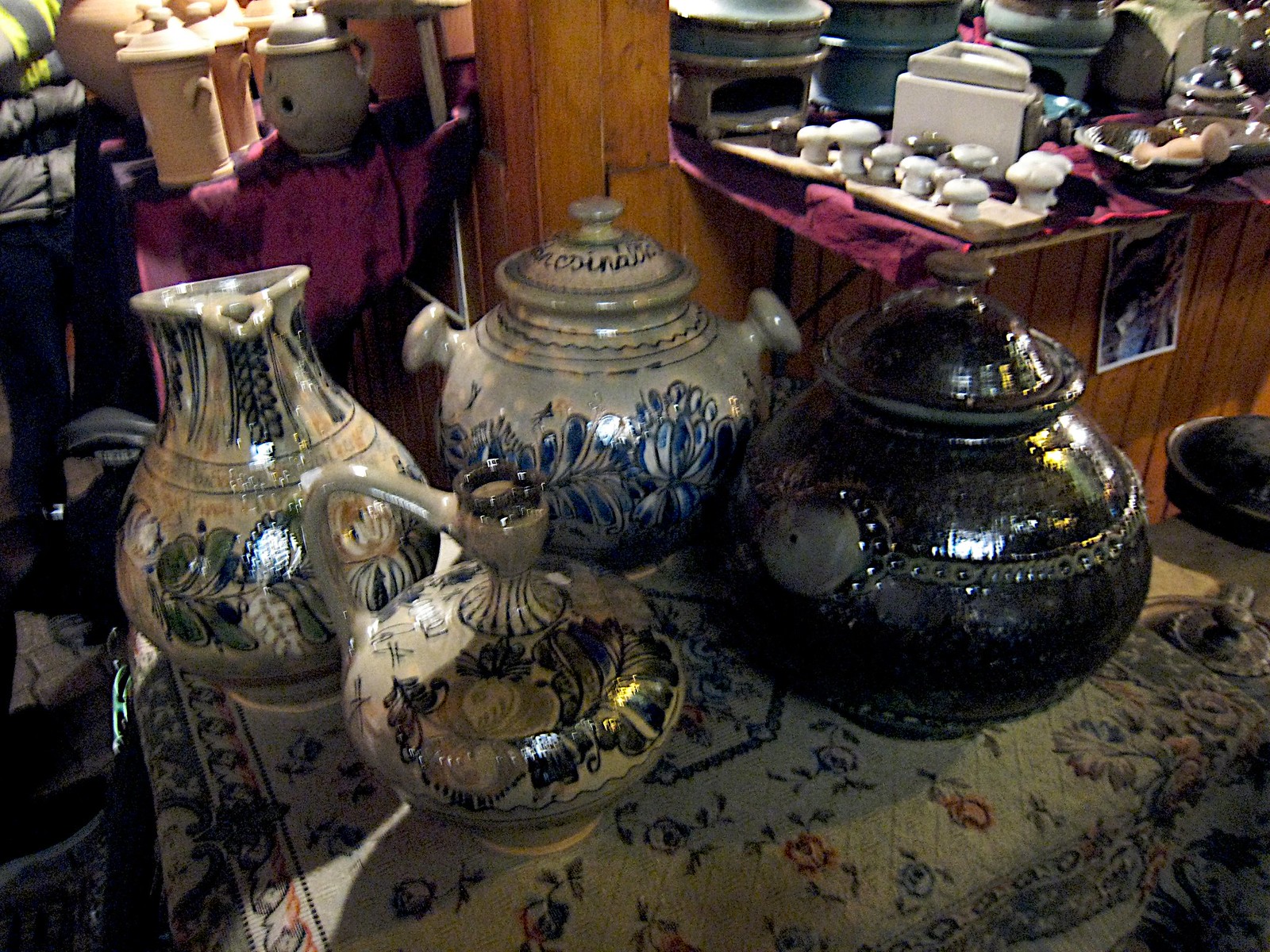The photograph captures a cluttered and crowded room, possibly an antique store, characterized by wood panel walls and multiple tables covered in vibrant textiles like purple cloths and a Turkish carpet. At the forefront sits a table draped with a colorful, intricate tapestry, upon which four ornate ceramic items take center stage. From right to left, there is a large black teapot with a lid, followed by a blue and white teapot adorned with intricate designs, a brown and green teapot, and a matching green and brown water pitcher. In the background, the scene is filled with an assortment of other ceramic vases and items, some appearing to be rare and expensive, with blue flowers and green foliage motifs. Piled on wooden counters, the ceramic collection presents a rich tapestry of history and craftsmanship, evoking the sense of an antique store brimming with treasures.